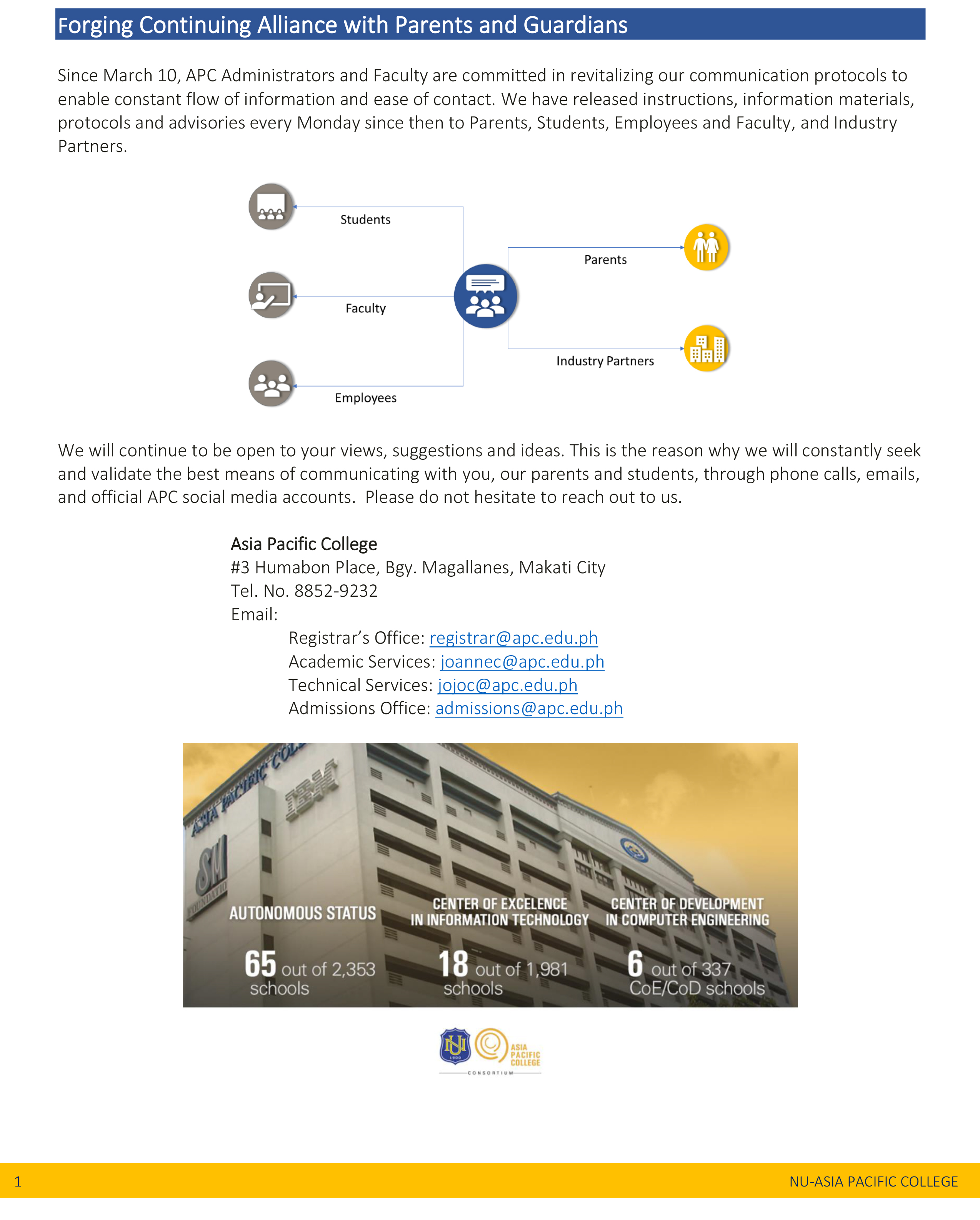The image features a dark blue header at the top with white text that reads, "Forging continuing alliance with parents and guardians." Below the header, the background transitions to white, displaying black text that states, "Since March 10, APC administrators and faculty are committed to revitalizing our communication protocols to enable constant flow of information and ease of contact. We have released instruction, information materials, protocols, and advisories every Monday since then to parents, students, employees, and faculty and industry partners."

Beneath this informative paragraph, there is a graphical representation. At the center of the graph, a blue circle is depicted, surrounded by smaller circles connected by lines. On the left side, the smaller circles are gray and are labeled from top to bottom: "Students," "Faculty," "Employees." On the right side, the smaller circles are yellow and are labeled: "Parents," "Industry Partners." 

At the bottom of the illustration, additional text conveys the organization's commitment to engagement: "We will continue to be open to your views, suggestions, and ideas. It is the reason why we constantly seek and validate the best means of communicating with you."